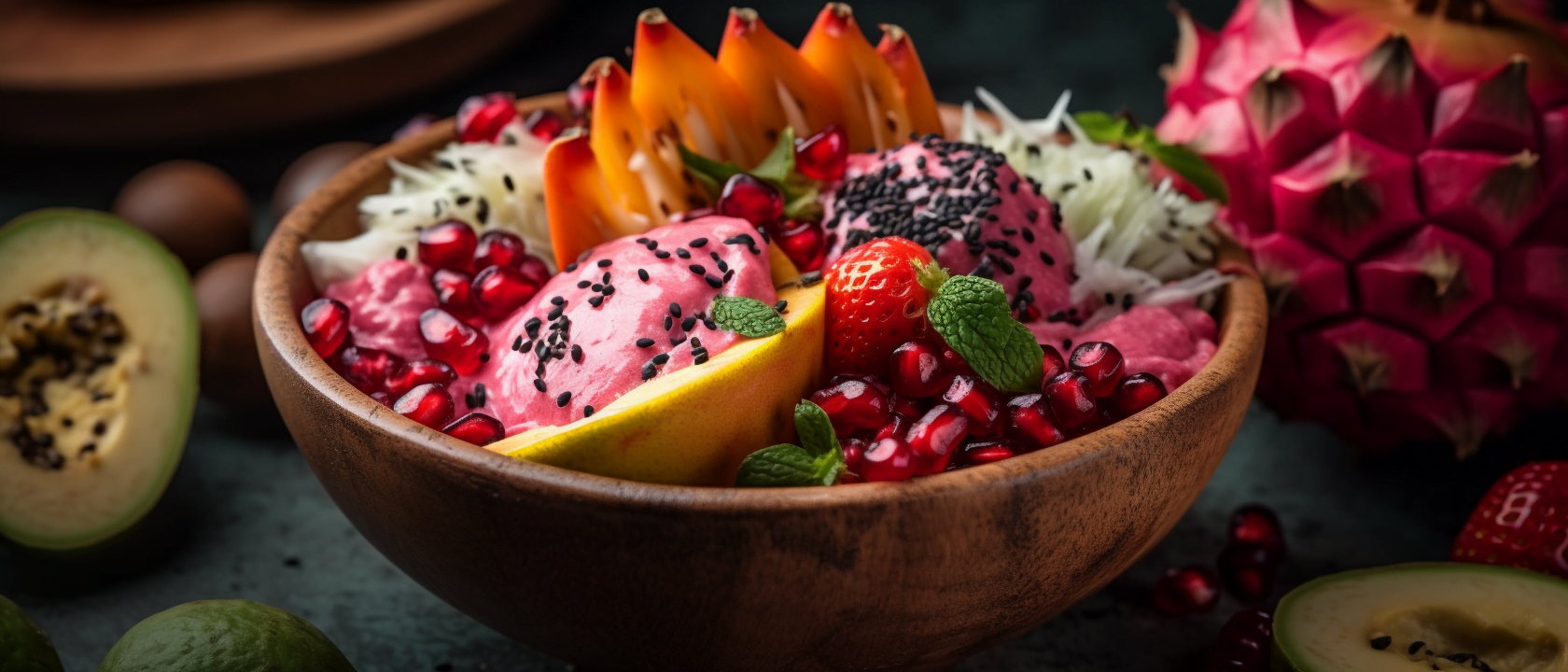A captivating photograph features a wooden bowl set on a dark surface, illuminated with focused lighting that highlights the bowl's contents while leaving the surroundings dim and moody. The bowl, the centerpiece of the image, brims with a variety of colorful fruits. There are strawberries, cranberries, dragon fruit, and an assortment of white-colored fruits, potentially including slices of mango or papaya. The vibrant mix inside the bowl displays a palette of pink, orange, red, and green hues. Surrounding the bowl and within the frame of the image are additional dragon fruits and avocados, adding to the exotic and abundant feel. The scene presents a visually rich array of textures and colors, with scattered mint leaves and dark seeds completing the composition.